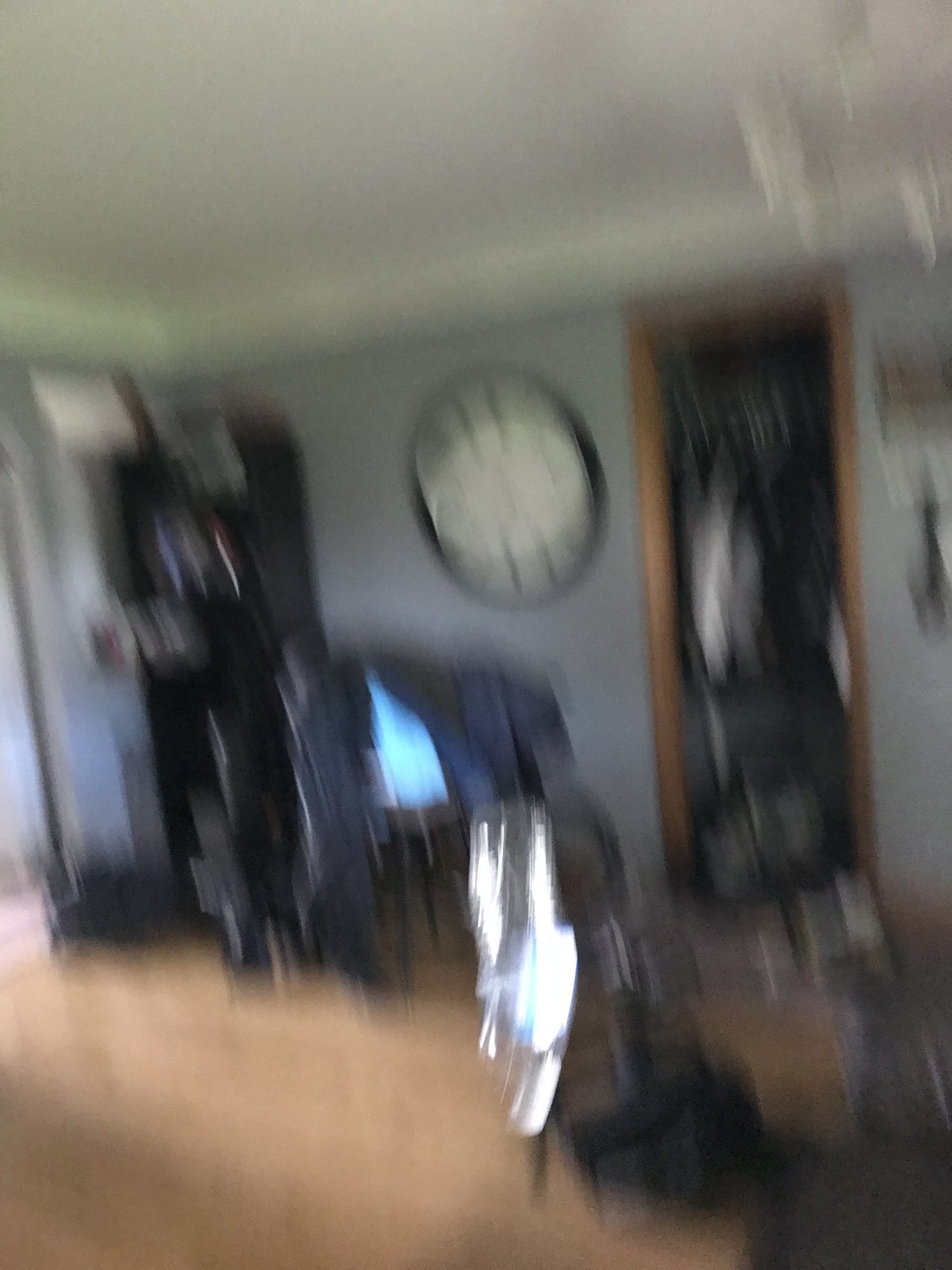The image depicts a blurred photograph of a living room corner characterized by white ceiling and wide white crown molding. The walls are a light gray with a hint of periwinkle blue, accentuated by a light brown hardwood floor. Dominating the center of the image is a large black and white clock with bold black numerals. To the left of the clock is a tall, dark bookshelf or display shelf, which is positioned near the room’s corner. Adjacent to this corner is a doorway, framed in brown wood, which appears to lead to a closet with clothes hanging inside. To the right of the clock, the wall extends to another doorway. Additionally, there's a peculiar structure on the bottom right corner of the image, featuring a dark circle, a silver rod, and a square of silver. The room is also illuminated by a bright blue light emanating from what seems to be a monitor or TV, casting a vibrant hue across the space.